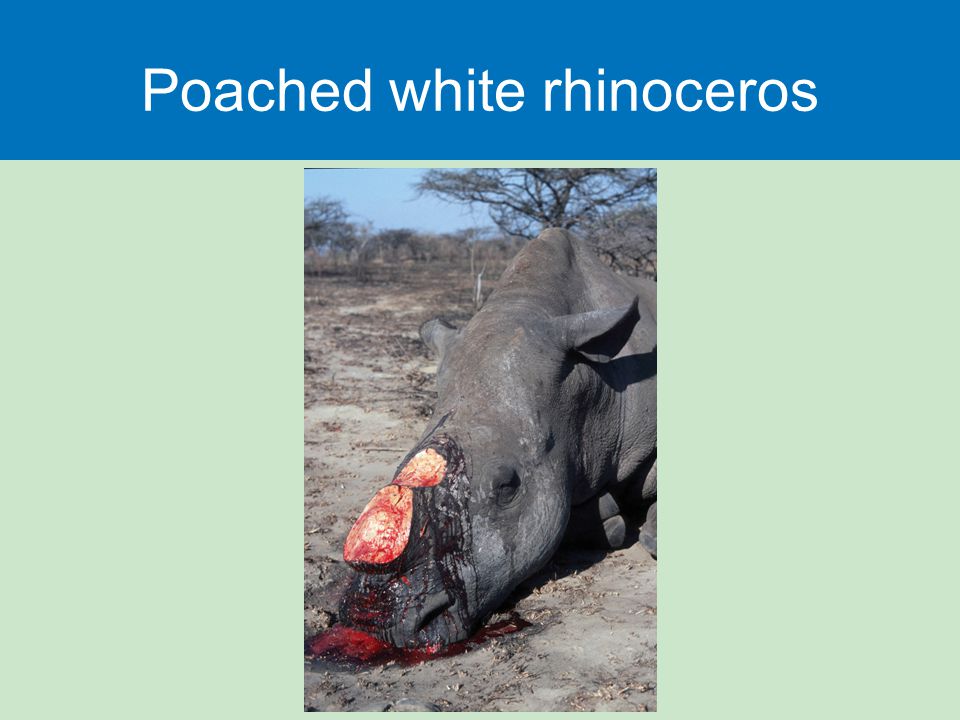The image titled "Poached White Rhinoceros" features a tragic scene of a dark gray rhinoceros lying lifelessly on a dusty tan and gray ground. Both of its horns have been brutally sawed off, leaving bloody stumps. Streams of red blood trickle down the animal's face and pool on the dirt below its head, intensifying the sadness and brutality of the scene. The rhino's eyes are closed, and although it isn't explicitly clear if it is dead, the stillness and bloodied state suggest its lifelessness. The setting appears to be a barren savanna with sparse brown trees and sparse gray vegetation under a clear blue sky. The poignant image is framed by a blue banner with white text reading "Poached White Rhinoceros," set against a light green background.